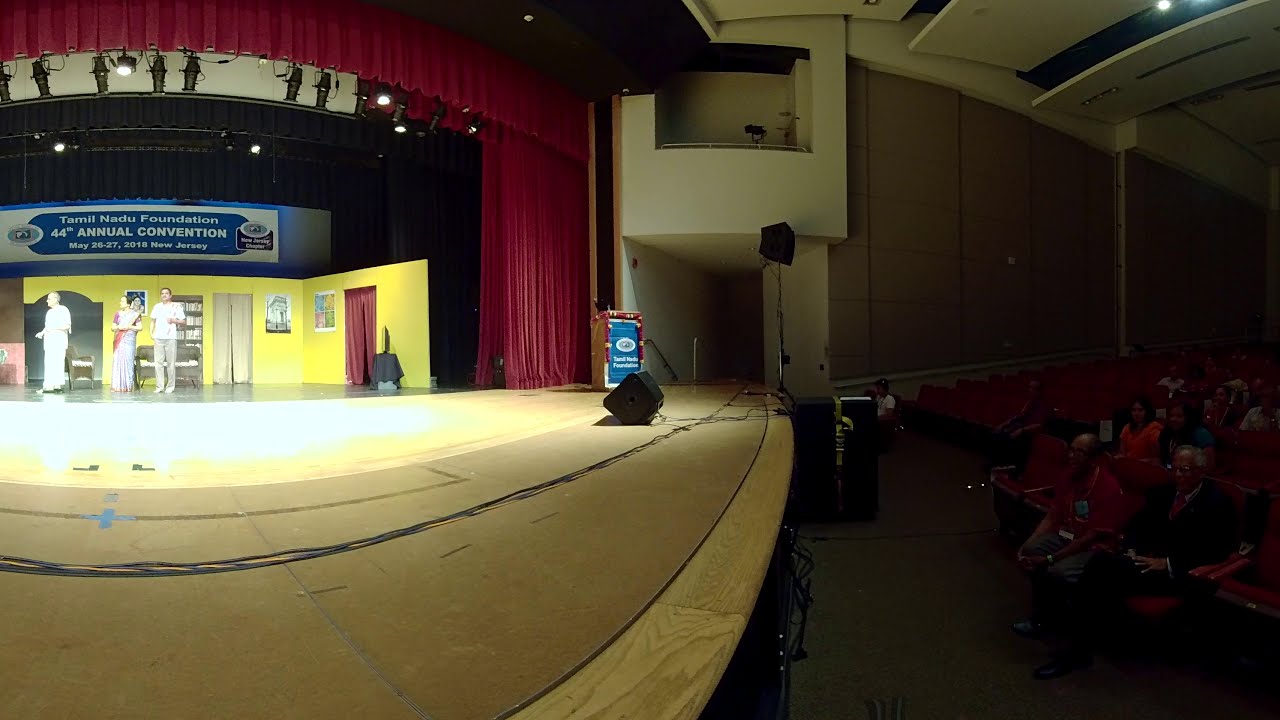The photograph captures an auditorium scene from the edge of a stage, viewed at a panoramic angle. The stage extends from the left side into the center of the frame, featuring a light tan wood base. Positioned on the stage are three performers—two men and a woman—each clad in white T-shirts and light-colored pants, standing within a meticulously arranged theater set. This set, resembling an interior room, boasts a yellow wall adorned with multiple doors and a bookcase, creating a homey atmosphere. Suspended above the stage is a prominent sign bearing the text "Tamil Nadu Foundation 44th Annual Convention, May 26th through 27th, 2018, New Jersey," in white against a blue backdrop. Overhead, deep red curtains and theater lights frame the scene.

On the right side of the frame, the darkened audience section features rows of red chairs occupied by viewers, predominantly black individuals, who focus intently on the performance. The walls around the seating area are a combination of tan and dark brown, with stage equipment and a speaker on a stand visible toward the back wall. High above, a cutout window resembling a booth may house a camera, enhancing the immersive documentation of the event. Thus, this image encapsulates both the engaging live performance on stage and the attentive audience, unified under the celebration of the Tamil Nadu Foundation's annual convention.